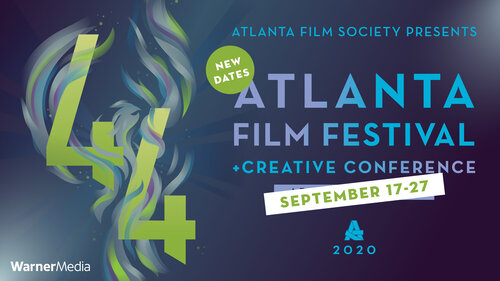This digital advertisement for the Atlanta Film Society's Atlanta Film Festival Creative Conference, held from September 17 to 27, 2020, features a design dominated by navy blue and various shades of purple, blue, powder blue, light purple, and army green. The left side prominently displays the number "44" in army green, surrounded by twirling flames in green, blue, and purple colors. To the right, important event details are spelled out in a mix of blue, powder blue, and light purple, noting the partnership with Warner Media, whose logo appears in the bottom left corner. The digital poster manages to incorporate a vivid palette to grab the viewer's attention within its relatively compact 3x3 format.